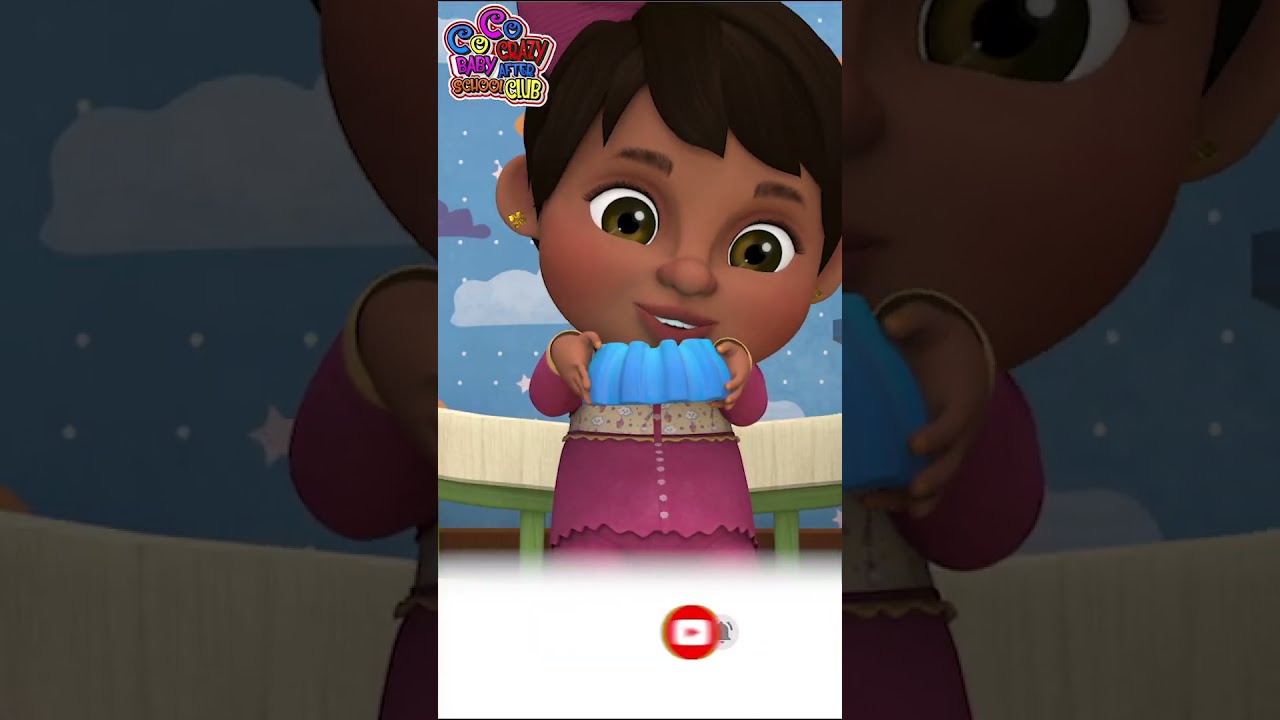This image is a detailed cartoon illustration of a young child with an exaggeratedly large head, adorned with short, dark-brown hair and big green eyes. The child is facing forward, slightly tilting their head to the right while holding an indeterminate blue item with ridges in both hands, as if poised to hand it to someone. The child wears a long-sleeved pink shirt and matching pink pants, complemented by a small, toothy smile. The background features a whimsical sky with various white dots, stars, and both white and dark clouds, akin to wallpaper art. A prominent watermark on top reads "Coco Crazy Baby After School Club" in a colorful mix of red, yellow, purple, and brown letters. Additionally, the lower part of the image includes the YouTube logo and a notification icon, suggesting that this may be a screenshot from a YouTube video. The entire image is framed by wide borders on either side, created from enlarged and grayed-out elements of the central illustration.